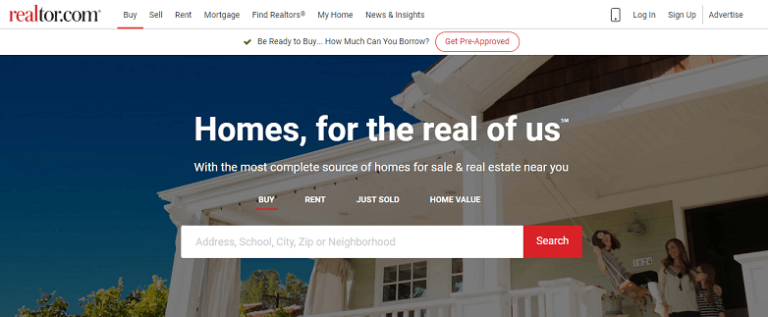A detailed screenshot from Realtor.com showcases an interactive and user-friendly interface designed for individuals seeking real estate information. At the top, navigational tabs allow users to explore different sections of the website, including "Buy," "Sell," "Rent," "Mortgage," "Find Realtors," "My Home," "News and Insights," alongside options to "Log In" or "Sign Up," and "Advertise." Currently, a red underline indicates the active "Buy" tab.

Below the navigation bar, a prominent message encourages prospective buyers to "Be ready to buy... How much can you borrow? Get pre-approved." This is accompanied by a central visual featuring a pristine white house, with people standing on its welcoming porch, embodying a sense of modern elegance. Overlaid text in bold white letters promotes "Homes for the real us," positioning Realtor.com as "the most complete source of homes for sale and real estate near you."

Further beneath, interactive tabs such as "Buy" (highlighted with a red line), "Rent," "Just Sold," and "Home Value" offer more browsing options. A comprehensive search box allows users to filter listings by address, school, city, ZIP code, or neighborhood. The conspicuous red "Search" button stands ready to refine property searches.

The backdrop of the image features a blend of serene blue skies and lush trees, enhancing the overall aesthetic and reinforcing the platform's commitment to offering idyllic home options.